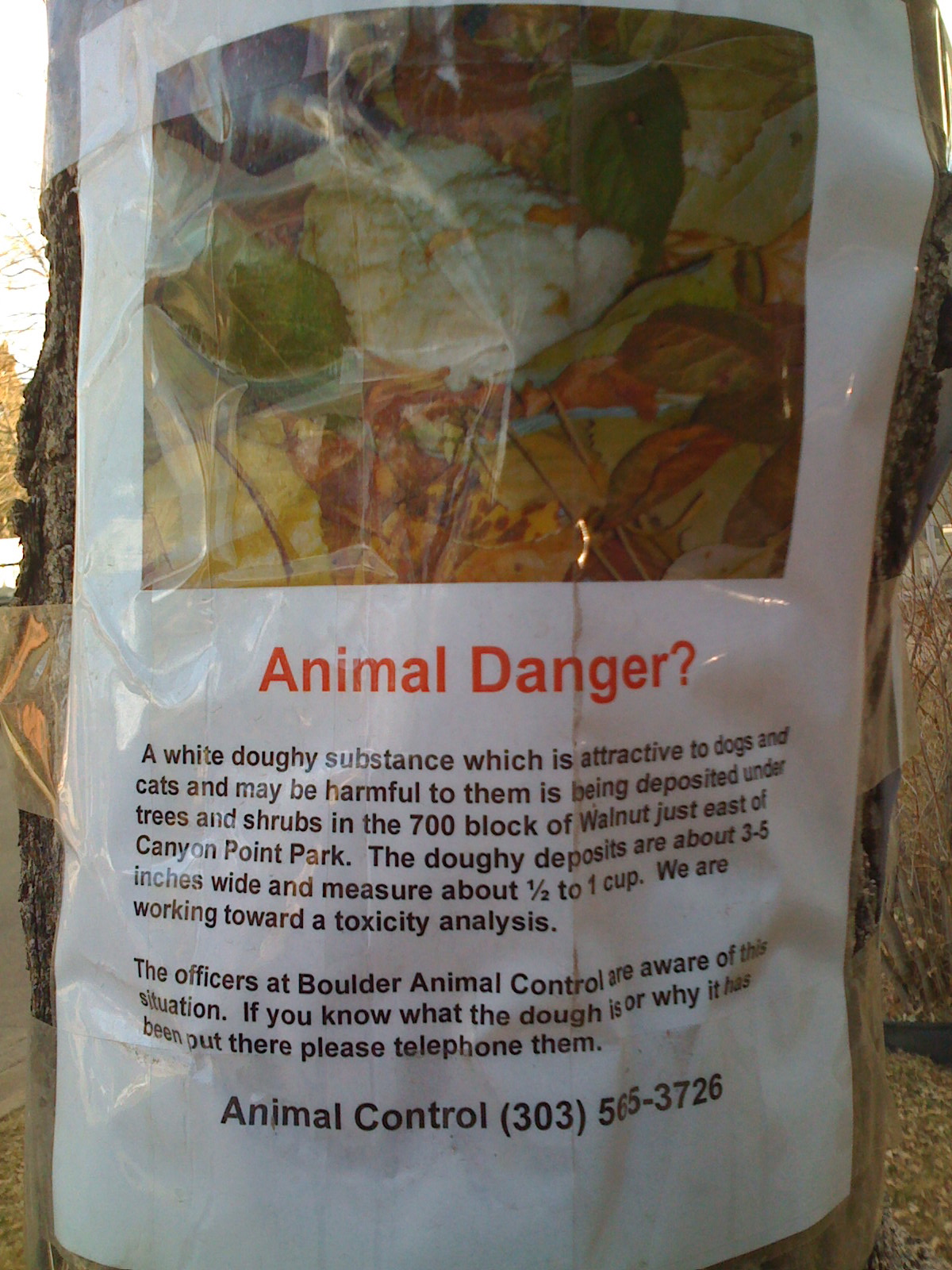The image shows a shiny, laminated pamphlet taped to a tree, making it appear rounded. At the top of the pamphlet is a blurry photograph, possibly of flowers or foliage. Beneath the photograph, the text "Animal Danger?" is written in prominent orange letters. The pamphlet contains a warning in white text on a black background, noting that a white, doughy substance, which attracts dogs and cats and may be harmful to them, has been found under trees and shrubs in the 700 block of Walnut, just east of Canyon Point Park. The doughy deposits measure about three to five inches wide and hold approximately half to one cup. The notice mentions efforts are underway for a toxicity analysis. The pamphlet further states that officers at Boulder Animal Control are aware of the situation and includes a request for information about the substance, alongside the Animal Control phone number, 303-565-3726.